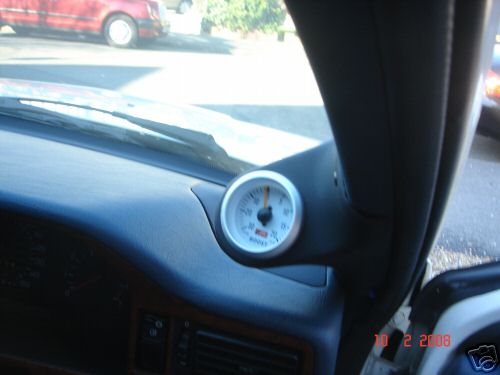This horizontal color photograph captures the interior view of a car from the driver's seat. The car door is open, revealing the edge of the vehicle, the door hinge, and part of the door itself. Prominently featured on the front passenger side of the black dashboard is a small, round, silver gauge with a red needle, though the details are too blurred to discern its exact function.

Through the windshield, one can observe the windshield wiper and the car hood, whose color appears ambiguous due to the glare from the sunlight—it might be white or light silver, but the light's intensity makes it difficult to determine precisely. Outside the car, a parking lot or street comes into view, populated by several vehicles. In the distance, a red car is vaguely visible, its position unclear as to whether it is parked or moving. Additionally, another car is visible through the open door, evidently idling with its taillights illuminated, indicating it is likely powered on.